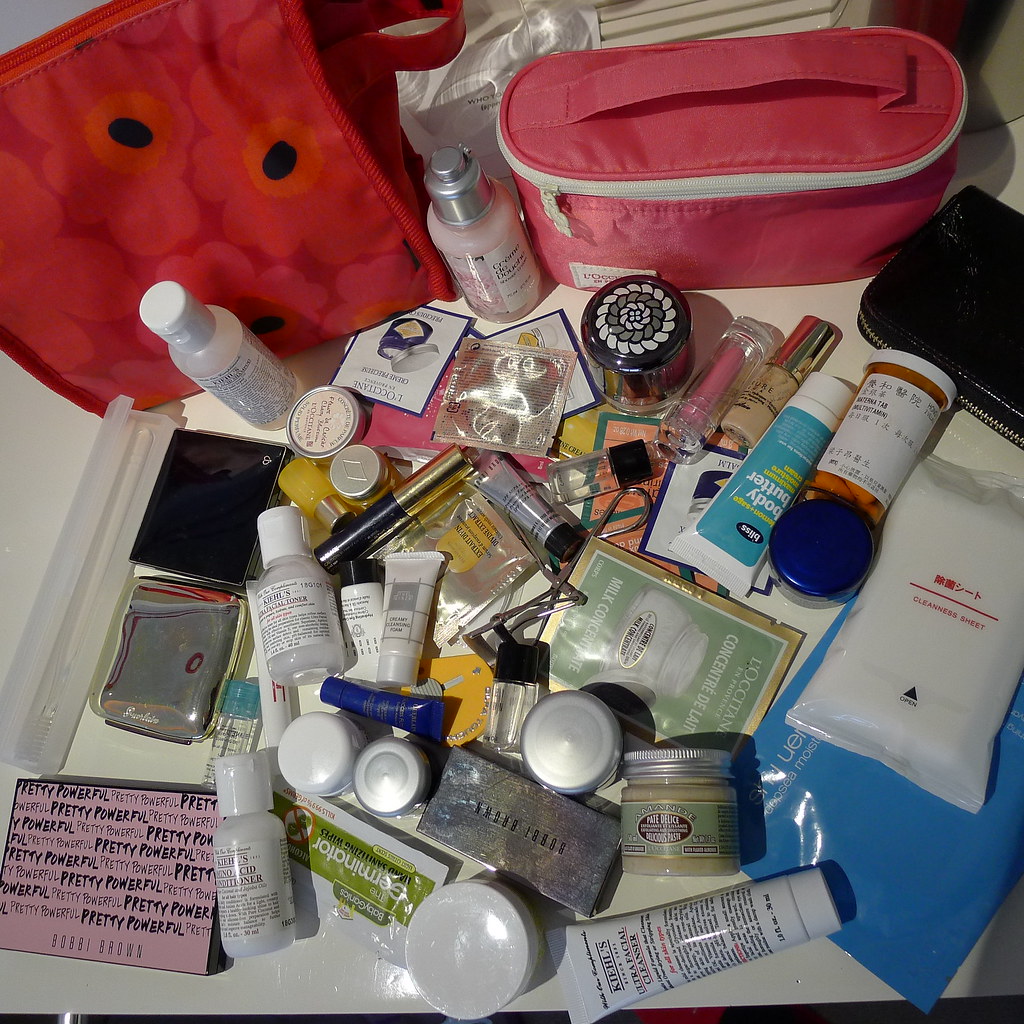This aerial photograph captures a cluttered yet colorful makeup counter set against a pristine white table. At the back, two large pink makeup bags dominate the scene. The taller bag has a canvas texture, adorned with vivid flowers in various shades of pink, orange centers, and dark accents. The other bag is structured, zipping fully around, showcasing a pink-toned body with a white contrast and a convenient pink handle on top.

A sliver of a black leather wallet can be seen peeking amongst the beauty chaos. The array of products sprawled across the table tells a story of diverse routines and preferences. Small bottles of skincare stand upright, alongside an assortment of product samples and essentials. The table also houses medications, a tub of body butter, and a signature Kiehl's cream, hinting at a diligent skincare routine. 

Not to be overlooked, a pack of makeup wipes lies ready for use, ensuring quick and efficient cleanup. A clear, travel-friendly toothbrush container signifies attention to hygiene, suggesting someone who is always ready to hit the road while keeping their essentials meticulously organized and protected.